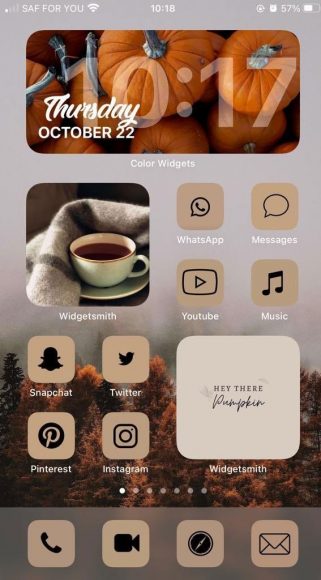This image, likely taken from a smartphone, showcases an autumn-themed home screen adorned with colorful widgets designed for the fall season. At the very top, the screen displays "SAF for you," followed by the time, 10:18, situated in the center along with a battery icon indicating 57% power on its right. Just beneath this, the date is noted as Thursday, October 22nd, 10:17. 

Prominently featured are a series of vibrant widgets: directly below the date, a "Widget Smith" displaying a cozy cup of coffee. The screen is dominated by various widgets in similar brownish hues, contributing to the seasonal aesthetic. On the right-center, app widgets for WhatsApp, Messages, YouTube, and Music are organized. To the left below, additional app widgets for Snapchat, Twitter, Pinterest, and Instagram are neatly aligned.

Further down, another "Widget Smith" features a welcoming message "Hey There Pumpkin," displayed in a grayish square. At the very bottom of the screen, quick-access icons are available for essential functions such as making a phone call, starting a video call, browsing the internet, or checking email.